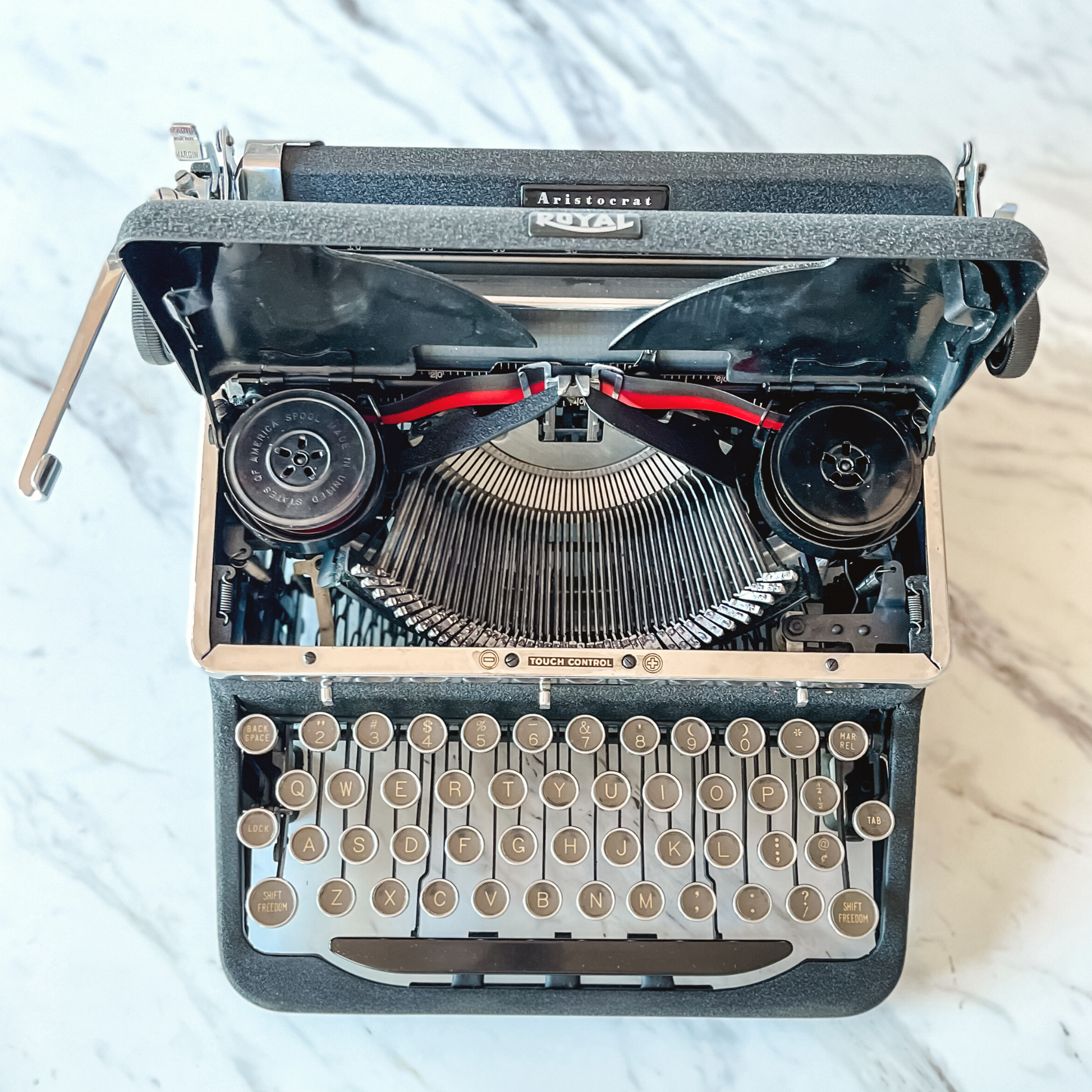This is a square-format color photograph that looks down on a vintage Royal typewriter placed on a white Carrara marble surface. The typewriter's front lid is lifted, revealing its intricate internal mechanics. Prominent in the view are the ribbon spools on both the right and left sides, holding a black and red ribbon that stretches across the center. A fan-shaped semi-circle with silver arms, each with raised letters, is displayed prominently at the bottom. Below them, the keyboard features individual keys with gold surfaces and white characters. The dark brown space bar spans the bottom of the keyboard. Additionally, the typewriter has a return carriage lever located at the top left and a small black label with the Royal logo on the edge of the lifted lid. This image exemplifies photographic representational realism, capturing in detail the vintage mechanism used before the advent of computers for typing documents and reports.